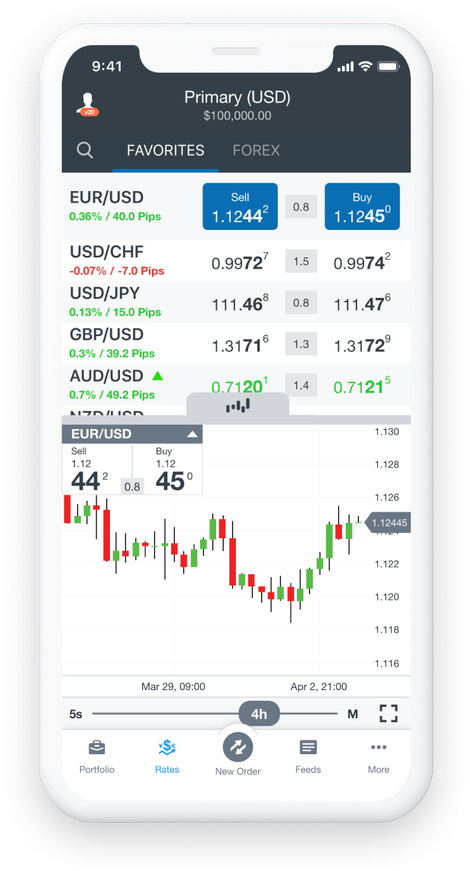### Descriptive Image Caption:

A close-up view of a smartphone screen displays detailed financial and trading information. The smartphone's edges are slightly blurry, possibly due to a focus on specific content. At the top of the screen, the status bar shows "12:41 PM," indicating full signal strength, Wi-Fi connection, and a fully charged battery. 

A primary financial balance of "$100,000 USD" is prominently displayed. Below this, a series of trading figures and currency pairs appear, offering detailed metrics:

- EUR/USD: 0.3%, 48 pips, showing rates from 1.1244 to 1.1245.
- USD performance: -0.07%, -0.97 with rates at 0.9872.
- GBP/USD: 0.3%, 39.2 pips, rates from 1.3171 to 1.3172.
- AUD/USD: 0.7%, 49.2 pips, rates at 0.7120 to 0.7121.

A section labeled "Sell" for EUR/USD shows rates at 1.12. 

The interface includes tabs for reverb settings ranging from 5 seconds to 4 hours and portfolio management options such as rates, new order, and fees. This setup seems to be part of a detailed financial trading app, allowing users to manage their investments and track market movements in real-time.